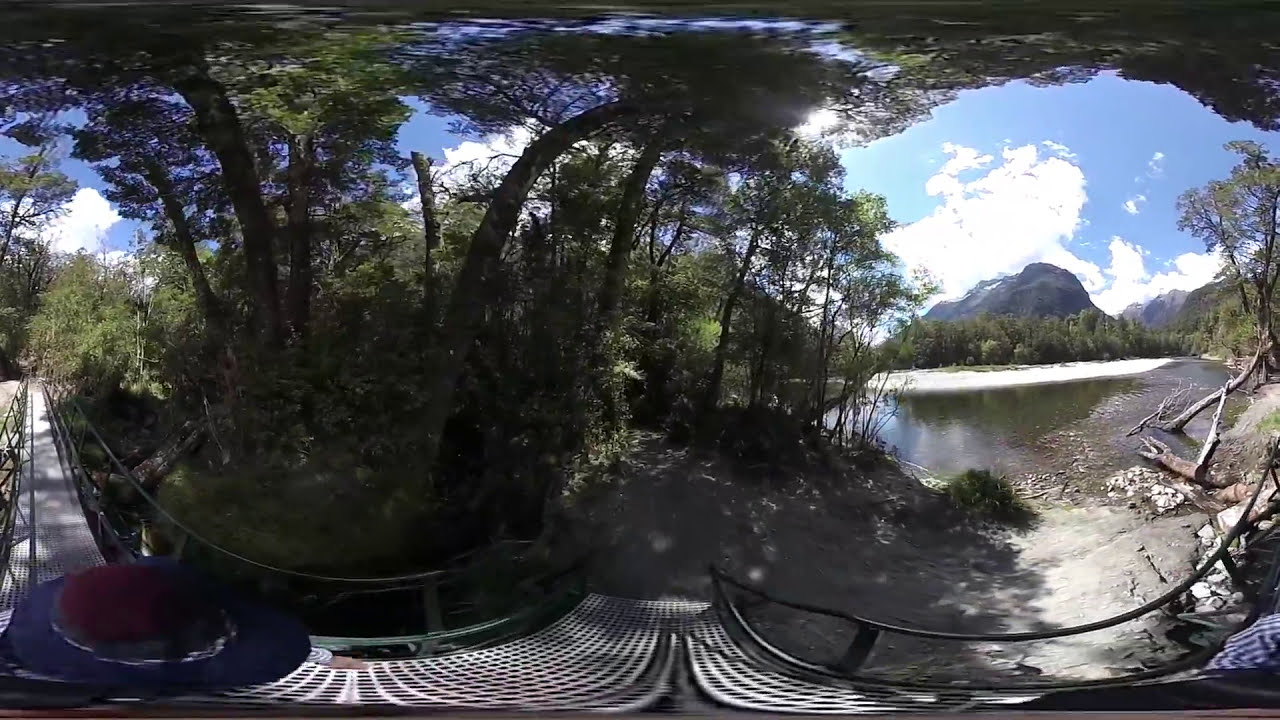The photograph captures an expansive and vibrant outdoor scene, presented in a panoramic view with a fisheye lens. Dominating the center of the image, a lush patch of tall, slender green trees with dense foliage stretches upwards, partially shading the area. Surrounding this greenery, a winding walkway begins from the left, curving gracefully around a small hill before descending towards the right, ultimately leading to a rocky, gray shoreline scattered with broken branches and logs. Along the path and flanking the trees, railings provide a sense of structure and direction.

To the right of the walkway, a serene body of water, likely a lake, reflects the day's brilliance. The shoreline there is dotted with bare, weathered wood and features sandy areas merging into the stony edge. Further back, the landscape is framed by imposing, dark gray rocky mountains, their peaks speckled with patches of snow, reaching majestically upwards. Above, the sky is a vivid, clear blue, adorned with fluffy white clouds. The sunlight bathes the entire scene, accentuating the varied natural hues of dark green, light green, blue, white, gray, brown, and silver. This detailed and lively photograph vividly captures the essence of a bright, sunny day in a picturesque natural setting.